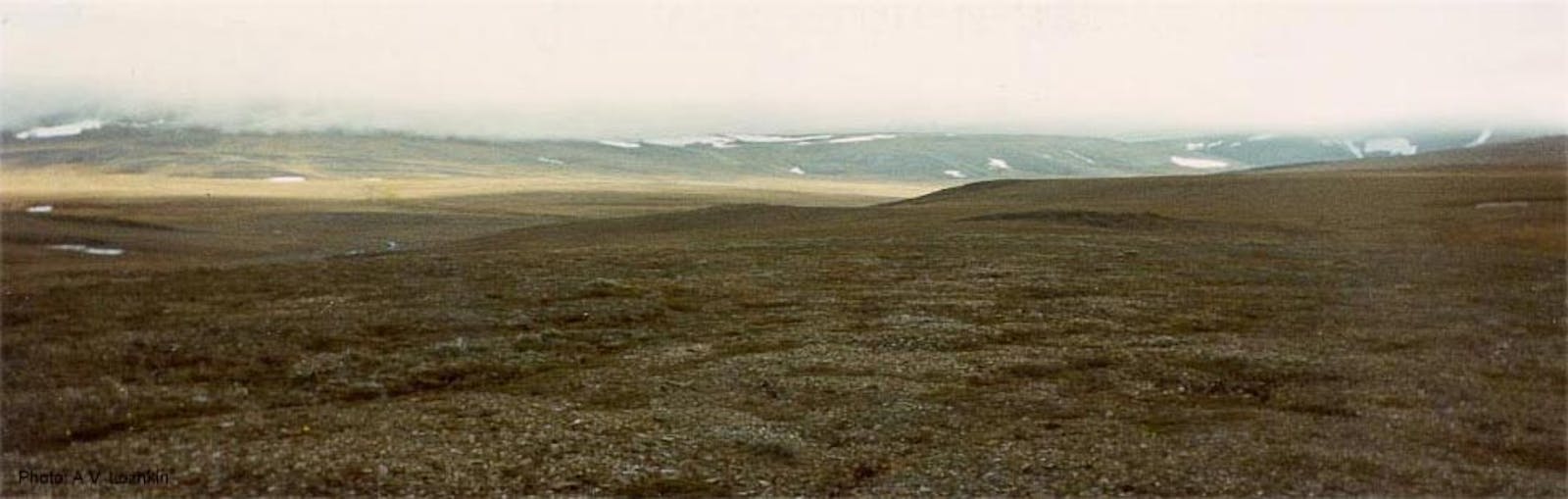This image captures a remote and scenic landscape characterized by a rugged mountainside in the foreground. The terrain in the front is uneven, with patchy areas of short, brownish grass. The ground features dark tones of brown and gray. As the landscape transitions into the distance, the color shifts to a sandy or muddy, light tan strip that runs horizontally across the image. This middle area has a distinct brownish-yellow hue. Beyond this, a set of rolling hills or mountains emerges, shaded in green and dotted with patches of white snow. The backdrop is veiled in thick, white fog which blends seamlessly with the cloudy, gray sky, creating a dull and overcast atmosphere that contributes to the remote and barren feeling of the setting.